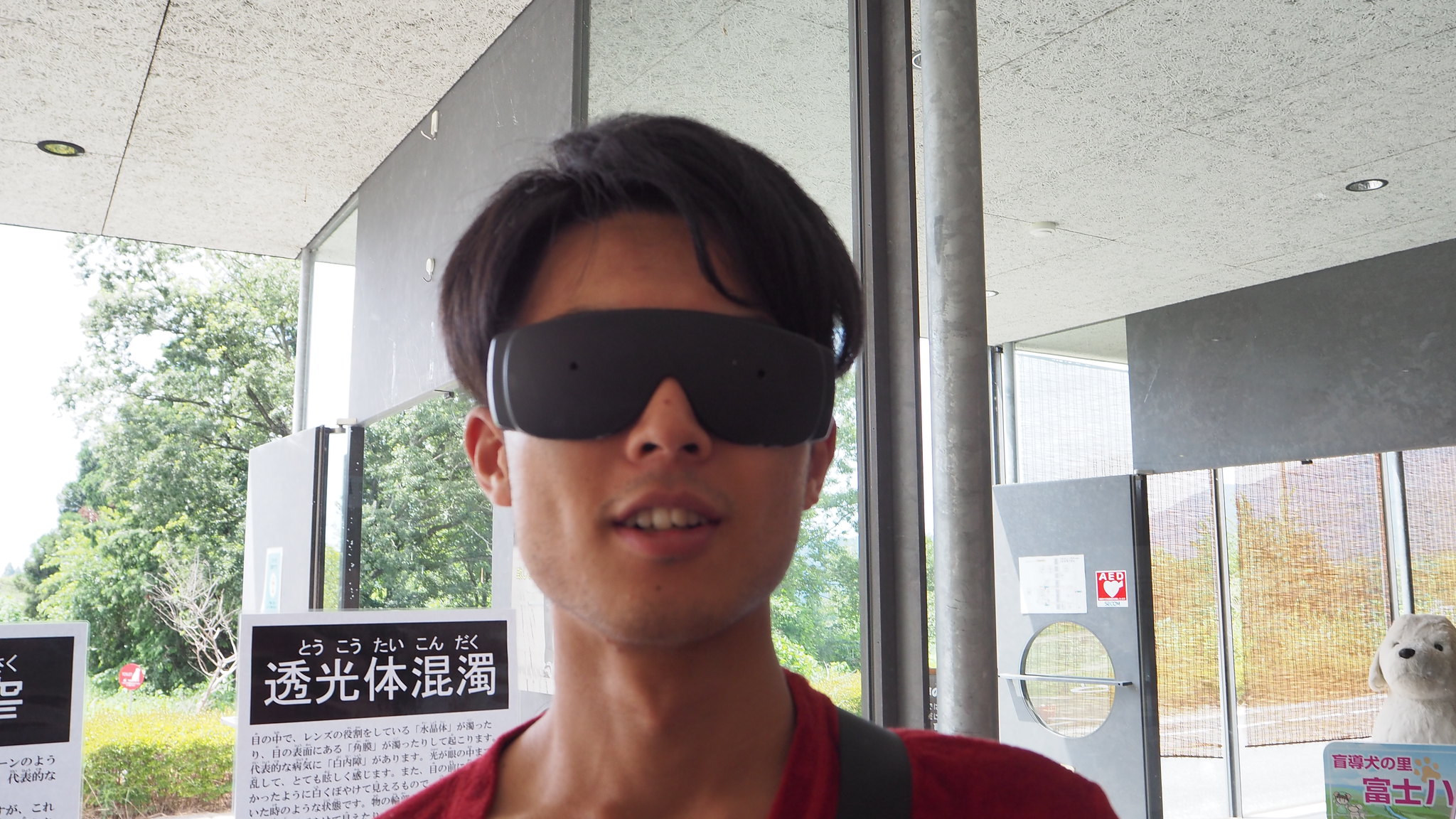This photograph captures a close-up of a man standing just outside of a shop with mirrored glass walls and a gray awning above him. The man, who appears to have Asian genetics with light olive skin, is dressed in a red shirt and has a black strap over his right shoulder, suggesting he is carrying a bag. He is wearing large, thick blackout sunglasses that resemble ski goggles, partially obscuring his eyes. His black hair is slightly wavy, parted to one side, and he has a faint mustache and a slight smile revealing his top teeth. In the background, there is a poster with black and white text in an Asian language, likely Japanese based on the included kanji and hiragana. Additional background elements include trees, a white teddy bear with pink Asian letters underneath it, and a bright sunny sign with pink writing. The scene is set on a sunny day, and the man is prominently positioned in the foreground, with only his head and shoulders visible.